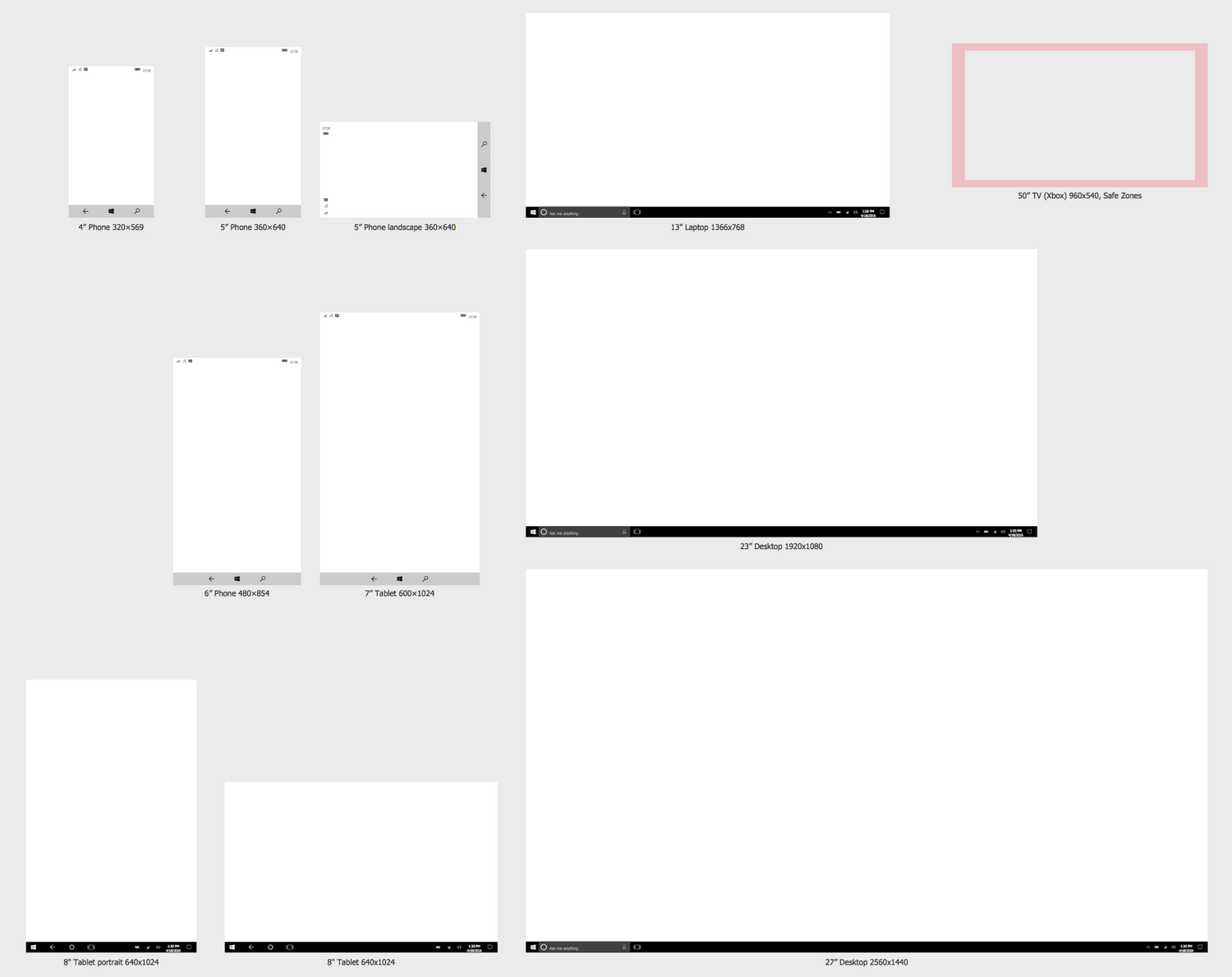The image features an array of boxes, each representing different screen sizes and device types against a gray background. 

In the top left corner, there are three different phone screens displayed, labeled as:
- 4-inch phone
- 5-inch phone
- 5-inch phone in landscape orientation

To the right of the phone screens, a 13-inch laptop screen is showcased.

Further right, a 50-inch TV screen is depicted with a red "Xbox" label.

Below the TV screen, a 23-inch desktop monitor is presented, designed in black and white.

To the left of the desktop monitor, various tablet screens are illustrated in different sizes. Notably, at the very bottom of this section, there are two types of 8-inch tablets:
- An 8-inch tablet in portrait orientation
- An 8-inch tablet in another form, both shown in white boxes

At the bottom right corner, a 27-inch desktop monitor is displayed, characterized by a white screen with a black line at the bottom.

Each box includes descriptive text detailing the screen dimensions and the devices they represent, illustrating the comparative sizes of these screens.